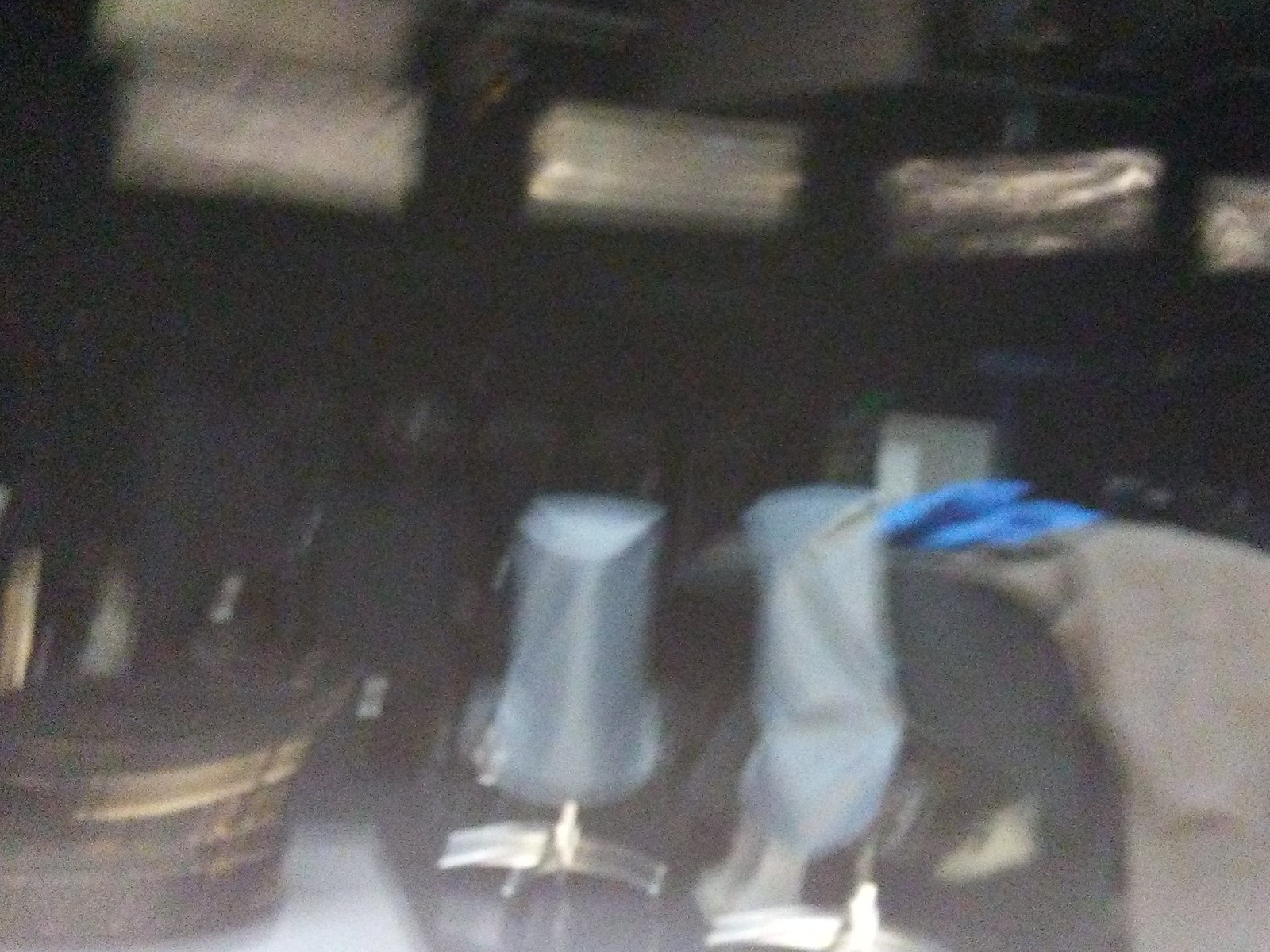The image is an extremely blurry and grainy interior shot with dull colors, making it difficult to identify specific objects clearly. In the background, there is a shelf holding grayish-white and gold-colored rectangular objects that seem to be made of fabric. Below the shelf, there appears to be a rack with clothes hangers. The foreground features a surface on which a brown wooden object sits on the left side, while to its right is a black object with two vertical, light blue rectangular items resting in the middle. There is also a gray section further to the right of this arrangement. Additionally, there seem to be office chairs covered in a loose-fitting blue fabric or plastic. These chairs have silver bases and are possibly positioned near a black table or surface. In the background, some silver-colored rectangular shapes hang, possibly from the ceiling or the wall. The image also vaguely shows rows of black folding chairs and an indistinct white object, potentially a desk or piano, with a blue tarp or cover on top. Overall, the image's poor quality and low resolution make it challenging to discern exact details.